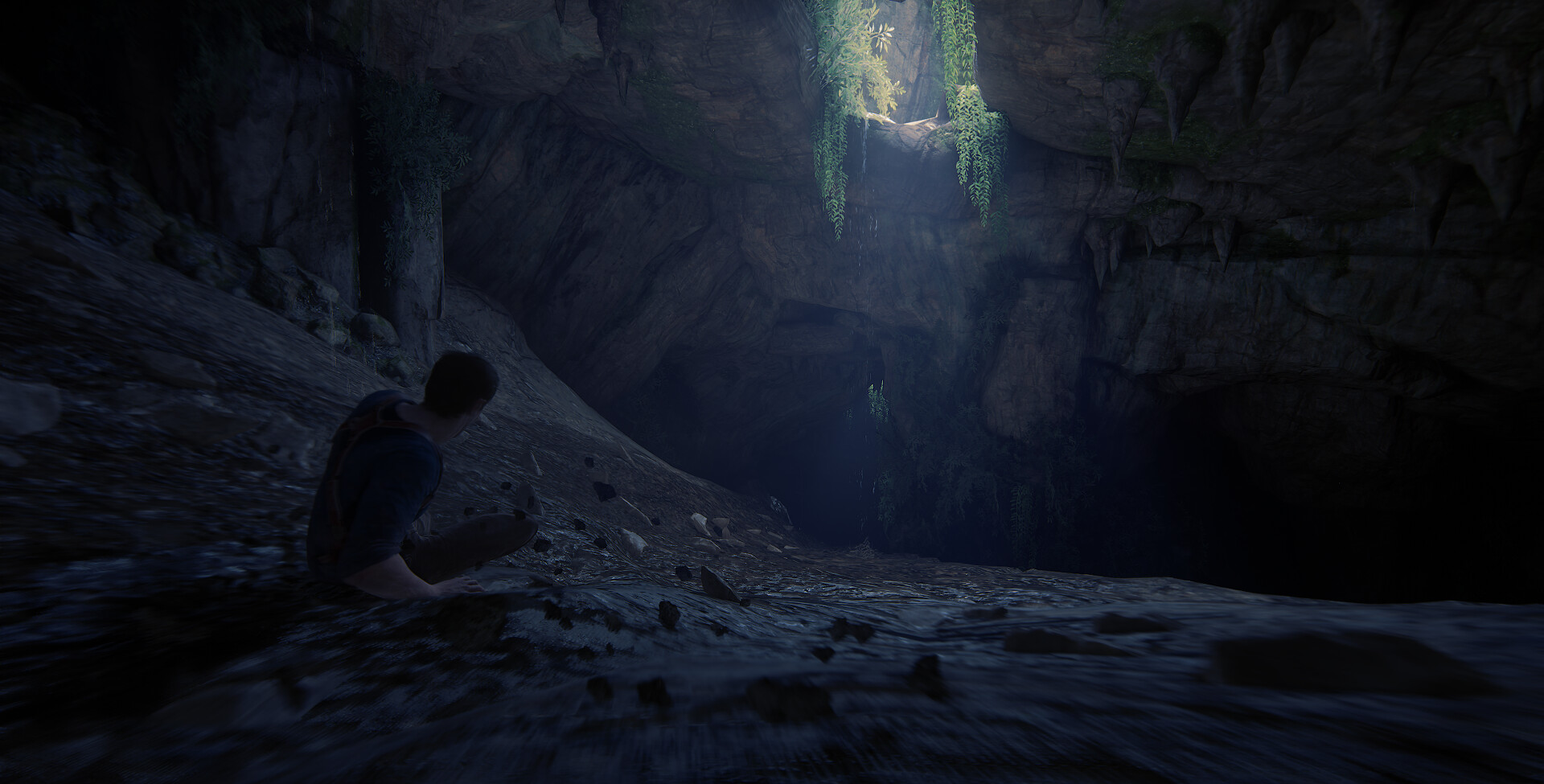A highly detailed rendering screen capture from a computer game shows an animated cave scene. The focus is on a character sitting cross-legged on the stony cave floor with their back towards the viewer. Visible are one arm, intricate details of the back of their head and neck, and their legs. The cave floor slopes upward to reveal rocky formations on the left. Directly ahead is a rugged wall of rock with a portion of the ceiling adorned with hanging stalactites. At the center top of the image, an opening allows daylight to stream in, illuminating patches of greenery growing around the entrance. The interplay of light and shadow within the cave, along with the detailed textures of the rocks and foliage, adds a lifelike depth to the scene.